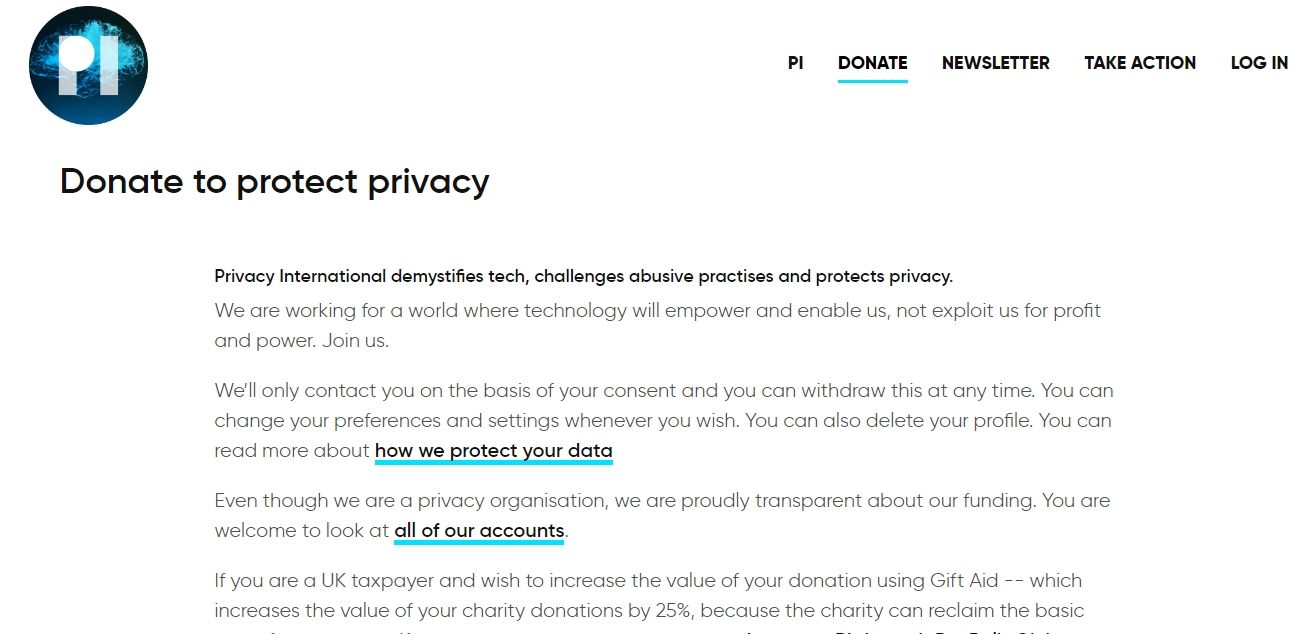The website's upper-left corner features a navy blue circle with a turquoise cloud-like design, overlaid with the white letters "P" and "I". To the right, in black capital letters, options for "PI," "DONATE," "NEWSLETTER," "TAKE ACTION," and "LOG IN" are listed, with "DONATE" underlined in turquoise. Beneath the emblem, a bold black text reads "DONATE TO PROTECT PRIVACY," followed by smaller black text stating, "Privacy International demystifies tech, challenges abusive practices, and protects privacy."

In gray letters, the text continues: "We are working for a world where technology will empower and enable us, not exploit us, for profit and power. Join us." The next paragraph states, "We will only contact you on the basis of your consent, and you can withdraw this at any time. You can change your preferences and settings whenever you wish. You can also delete your profile. You can read more about how we protect your data," with the latter phrase underlined in turquoise.

The subsequent paragraph asserts, "Even though we are a privacy organization, we are proudly transparent about our funding. You are welcome to look at all of our accounts," with "all of our accounts" underlined in turquoise. It adds, "If you are a UK taxpayer and wish to increase the value of your donation using Gift Aid, which increases the value of your charity donations by 25% because the charity can reclaim the basic..." Unfortunately, the rest of the text is cut off, leaving part of the message unreadable.